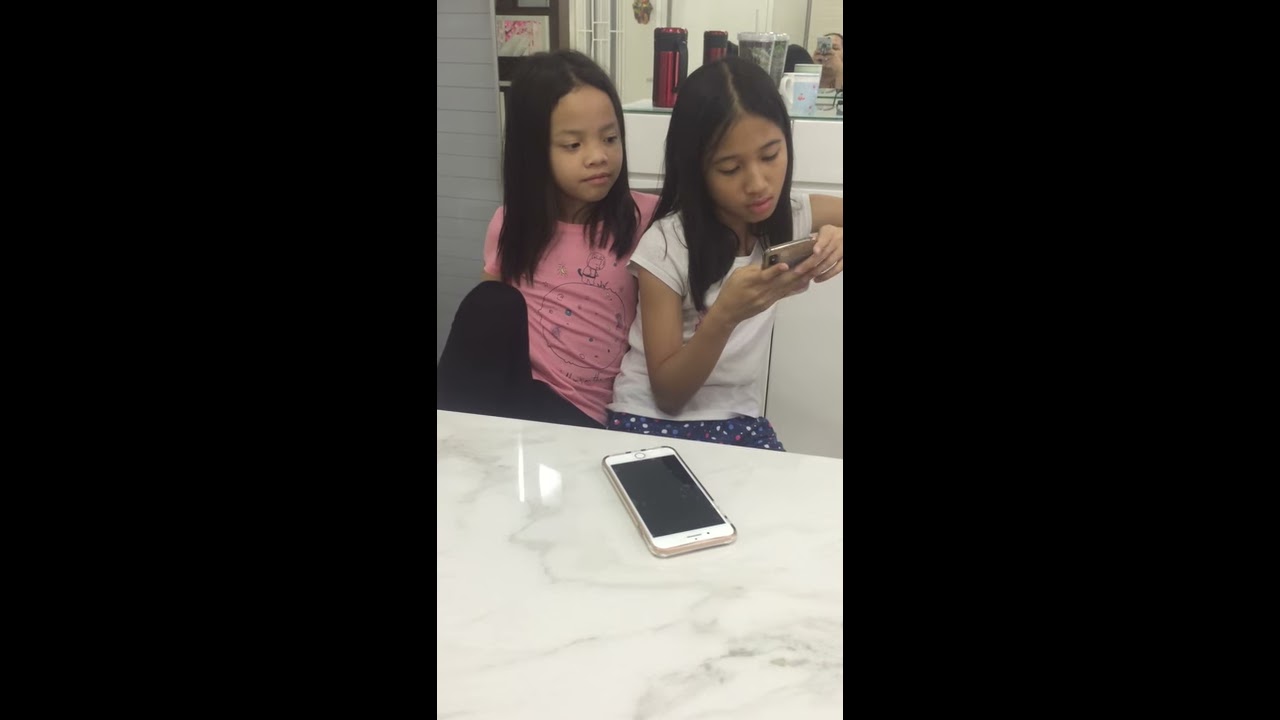In the center of a vertically-oriented image, two young girls are seated close together. The girl on the left wears a pink shirt and black pants, while the girl on the right is dressed in a white shirt and blue patterned pants. Both have long dark hair. The girl on the right is holding a cell phone with a white border and a black middle, and both are intently looking at it. Below them is a white table with another cell phone placed towards the girl on the right. In the background, between their heads, is a red thermos with black accents. In the top right corner of the image, a mirror reflects the head of a woman, likely their mother, taking the picture with her phone. The scene appears to be set in a kitchen, with a white counter visible behind the girls.